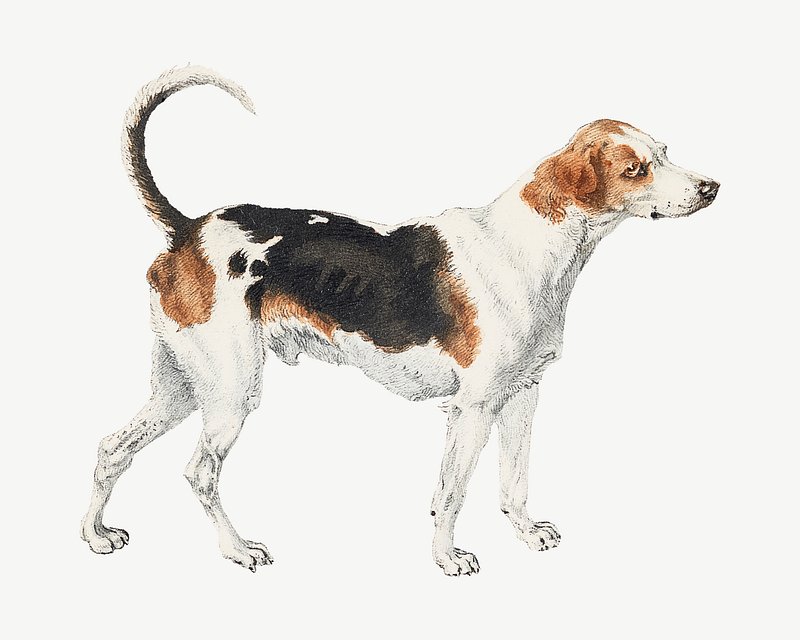This is a detailed illustration of a large dog, likely a hound mix with beagle-like features, set against a plain white background. The dog has a predominantly white coat with distinct brown and black markings. Notably, it sports brown patches around its face, particularly around the eyes and ears, and additional brown patches on its hind haunches. Black markings are prominent along the top of its curved tail, which ends in a hook-like shape that curls upwards in a friendly manner. The dog's ears are down, complementing its amiable expression. Its body is detailed with clear shading, showing black and brown spots scattered across its frame, and its nails are visible on its toes, adding to the meticulous detail of the illustration. The dog is facing to the right, appearing a bit slender, and conveys a neutral expression.